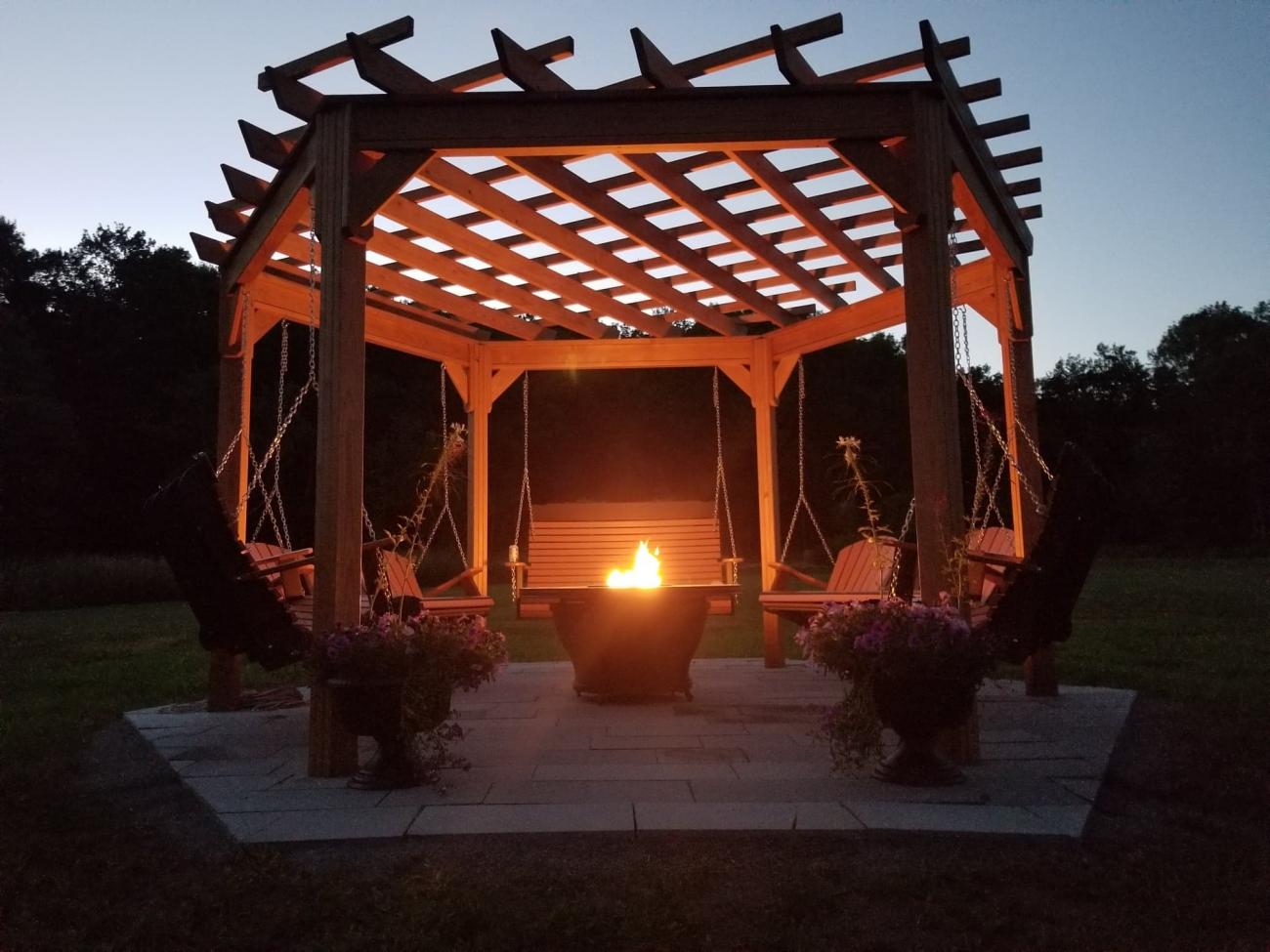In a professionally shot, full-color photograph taken just after sunset, a beautifully crafted outdoor gazebo becomes the focal point. The wooden structure features a roof made of crisscrossing wooden slats in a checker pattern, supported by large, sturdy beams. The gazebo houses at least three swinging benches - one two-seater and several single seats - all hanging from chains and crafted from reddish-brown wood.

In the center of the gazebo, there is a gas fire pit with a bowl-like design, emanating bright flames that illuminate the surrounding area. The gazebo is situated on an elevated stone-tiled platform, hexagonal or octagonal in shape, surrounded by lush green grass. Adorning the base of the wooden supports are two large stone plant containers overflowing with green vines and vibrant purple flowers.

Beyond the gazebo, the silhouettes of trees stand against a darkening sky, which still holds a light blue hue. The scene, clearly posed and staged, captures a moment of tranquil beauty just after dusk, with the fire pit providing a warm and inviting glow.